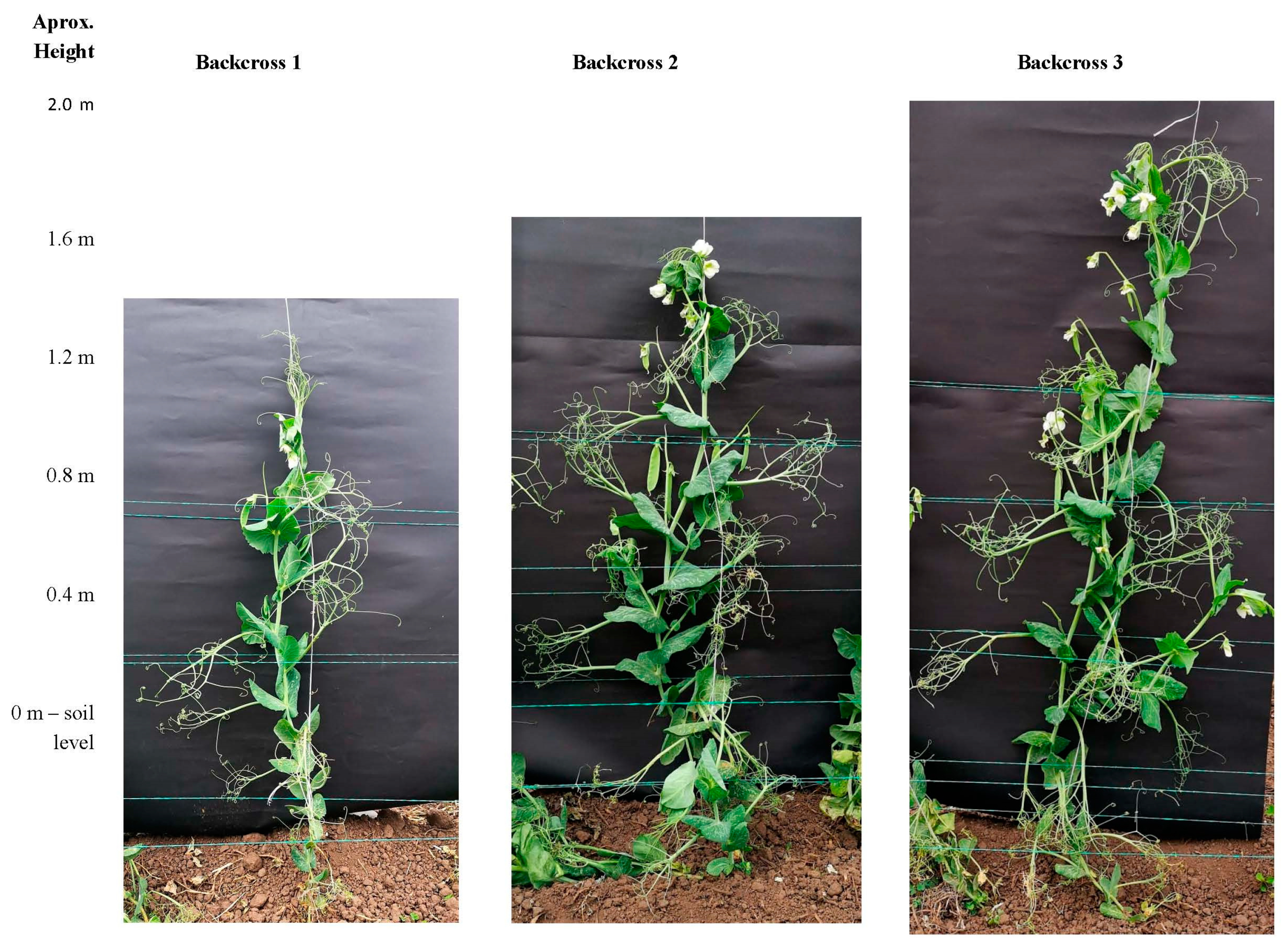The image is a composite of three photographs depicting the growth stages of a vine-like plant, each labeled "Back Cross 1," "Back Cross 2," and "Back Cross 3." Arranged sequentially from left to right, these photos illustrate the plant's progressive increase in height, resembling a bar graph. A scale on the left margin marks heights from 0 to 2 meters, with "soil level" indicated at the bottom.

In the first image ("Back Cross 1"), the plant reaches approximately 1.6 meters. It is primarily green with supportive strings vertically behind it. The second image ("Back Cross 2") shows the plant slightly taller at 1.8 meters, beginning to display flowers at the top. The third image ("Back Cross 3") depicts the plant at its tallest, reaching up to 2 meters, with a broader structure and more flowers, filling the entire vertical space of the frame. Each plant is rooted in brown soil, set against a gray background, with horizontal green strings providing additional support visible in all three images.